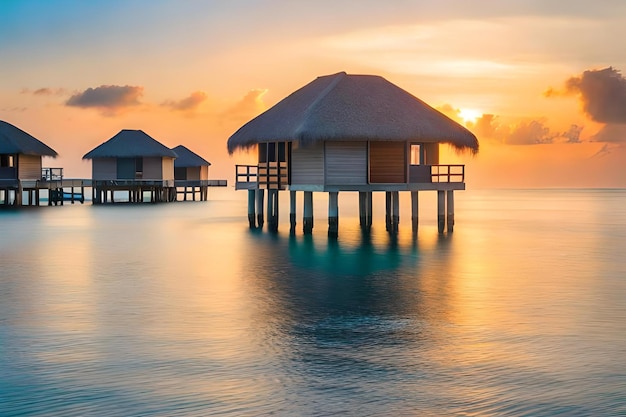This dreamy, idyllic photograph captures a tranquil tropical scene at sunset. The sky, painted in shades of orange, yellow, and blue, is partly veiled by wispy clouds, with the sun setting behind the main central hut in the foreground. Four thatched-roof bungalows, each square with small balconies, stand on stilts above calm water that reflects the serene hues of the sky. The central hut dominates the scene, while three smaller, interconnected huts with steps leading down into the water are to its left. The water, variegated in shades of yellow, green, and gray, adds to the peaceful ambiance, evoking a strong desire for a vacation in this picturesque and quiet setting.